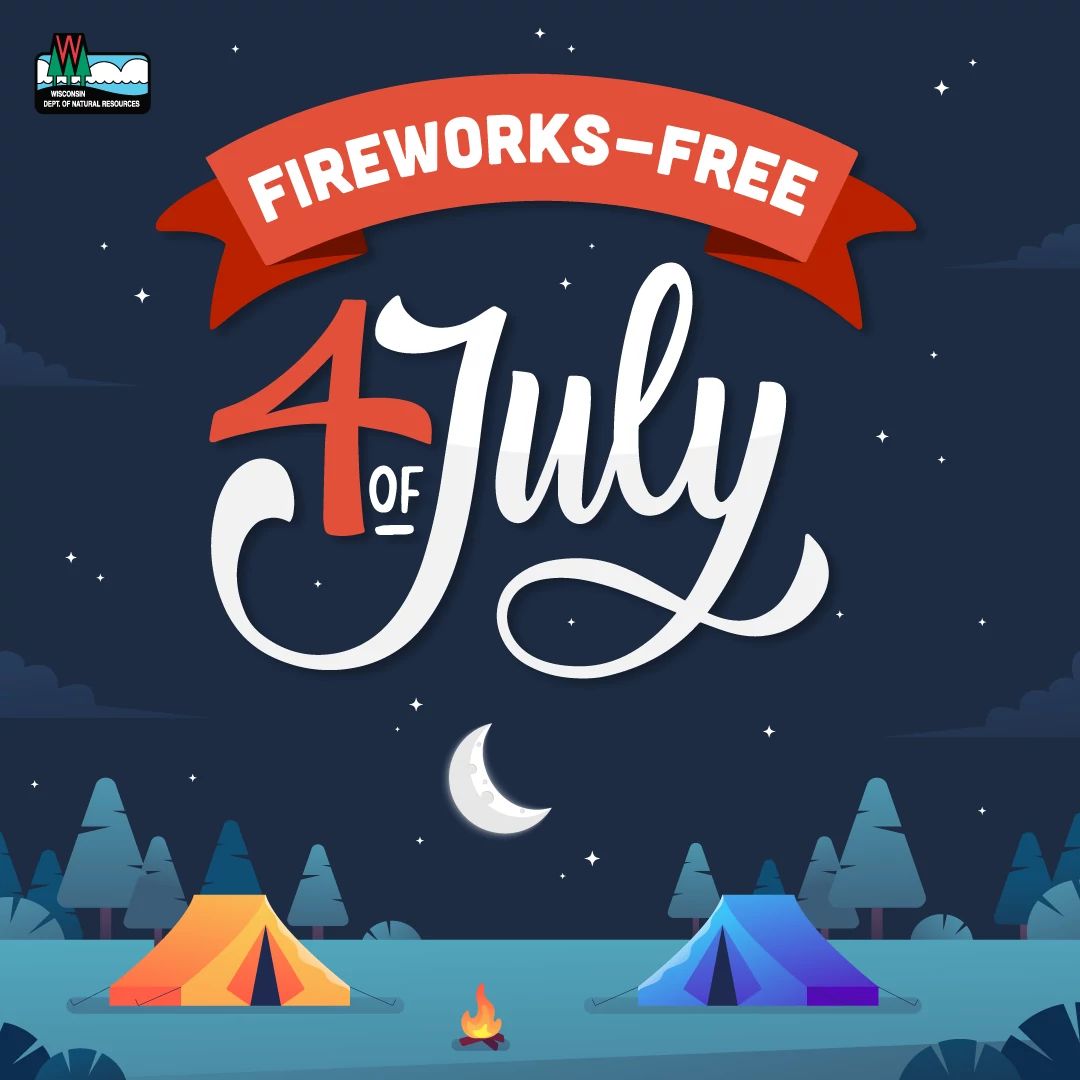The image is a cartoon-style advertisement for a fireworks-free 4th of July event, created by the Wisconsin Department of Natural Resources. It depicts a simple campsite scene with an orange tent on the left and a blue tent on the right, flanking a small, bright orange campfire. The tents and campfire rest on a flat, teal or green ground. In the background are stylized trees, represented as teal or green triangles with brown trunks. Above the campsite, the dark navy blue night sky is dotted with small white stars and features a bright crescent moon. At the top of the image is a large red banner with white text that reads "Fireworks-Free," while below this, in the center, large stylized red and white letters announce "4th of July," with "July" in an elegant cursive font. The top left corner of the image features a watermark of the Wisconsin Department of Natural Resources, depicting pine trees against a background of clouds.